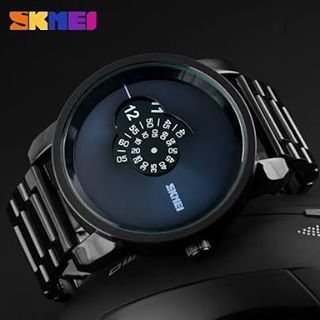This photograph features a Skamai men's dress watch showcased against a dark charcoal black background. The watch possesses a distinctive and sleek black design, complete with a flexible metallic band and a large, round face. The face of the watch transitions from black to dark gray and features a complex dial design. At the center, a circular black dial displays white numbers for seconds, while a semicircle at the top, containing more white numbers, marks the minutes. Above this is another semicircular shape with the number 12. The name "SKMAI" is prominently displayed in white text at the bottom of the watch face. Signifying its brand, the top of the advertisement displays "SKMAI" in vibrant, multi-colored letters: the S in orange, K in yellow, N in blue, E in purple, and I in pink. The watch is slightly tilted to the left, emphasizing its elegant and modern appeal.